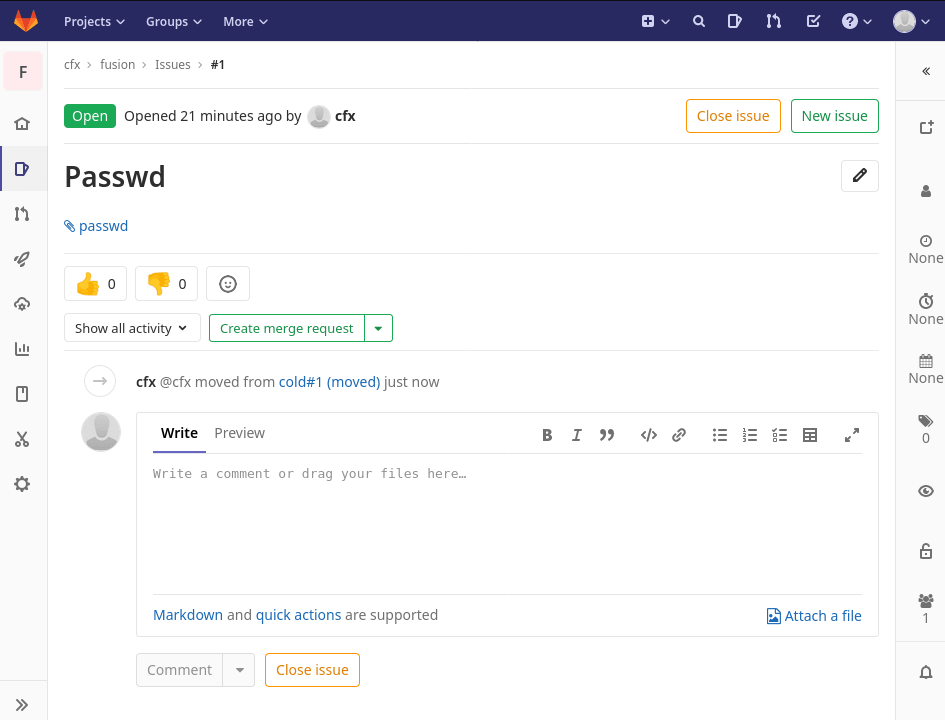**Caption:**

The image displays a website with a dark blue header featuring a two-tone fox head logo on the top left. Next to the logo are three expandable links labeled "Projects," "Groups," and "More," each followed by a downward-pointing arrow. On the right side of the header, there is a row of seven icons representing various functions such as a user profile, information, a checklist, and search.

The main body of the website is predominantly white, with very pale gray vertical margins on both sides. The left margin contains several icons in a vertical row: an "F" inside a pale pink square, a home icon, a coffee mug, arrows, a rocket ship, a cloud, a graph, a smartphone or date icon, scissors, and a gear icon for settings. 

The right margin features icons including a user profile, a clock with "none" underneath, an alarm clock with "none," and a calendar, indicating currently unscheduled activities.

At the top center of the webpage, text reads "CFX > Fusion > Issues > #1." Below this line, a green rectangle labeled "Open" is followed by text stating "opened 21 minutes ago by" accompanied by a user profile icon with "CFX" next to it. To the right, there are two buttons: "Close Issue" in orange and "New Issue" in green.

Further down, bold black text reads "PASSWD" with a small edit-pencil icon to its right. Beneath this, a blue paperclip icon appears next to smaller blue text "password PASSWD." Another horizontal line separates this section from yellow thumbs-up and thumbs-down emojis, each in a rectangle with a count of zero, and a yellow smiley face icon. Underneath, text says "Show all activity" with a clickable option, and "Create merge request" in green with an expansion arrow.

The text "CFX at CFX moved from cold #1 (moved just now)" is shown in gray and blue. The bottom section resembles an email editor with options to write or preview content, currently in write mode. Editing options include bold, italics, and various alignments. The placeholder text reads "Write a comment or drag your files here..." with a note at the bottom stating "Markdown and quick actions are supported," both clickable links. In the bottom right, there's an icon to attach a file, depicted as a photo with a turned-over corner.